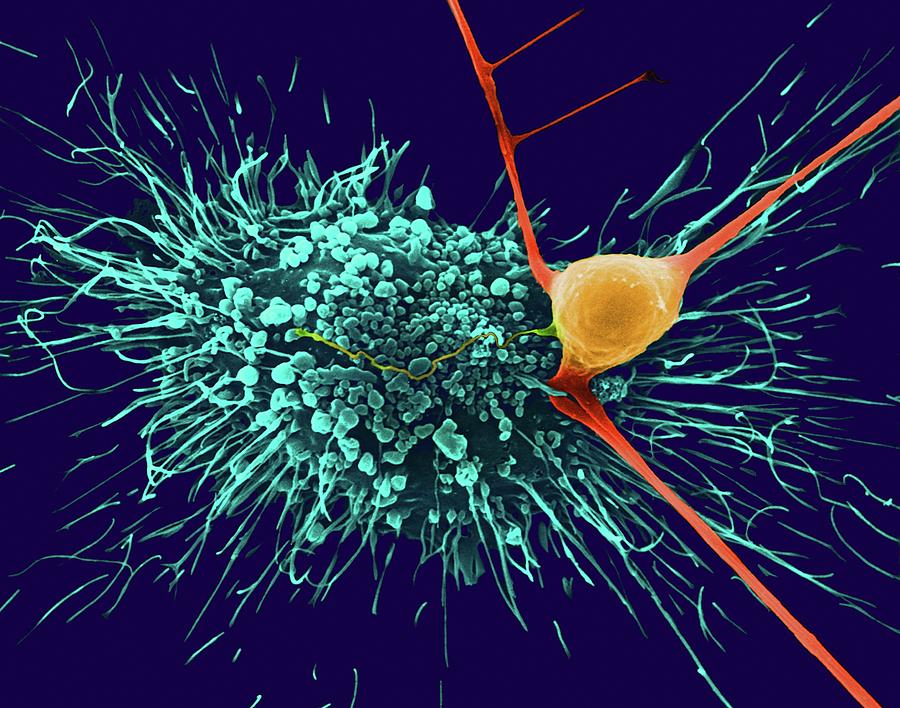The image appears to be an artistic rendering of a microbial structure, possibly depicting some form of bacteria being interacted with by another entity. The central focus is a teal, aquamarine-colored organism adorned with numerous hair-like strands extending outward. This organism has a blobular form and is set against a dark blue, almost purplish background, providing a stark contrast that highlights its features. To the side, an orange, globular object is present, characterized by three vein-like, reddish-orange structures reaching towards the central organism. This secondary structure also shows spiked extensions and appears to be engaging with the teal organism, suggesting a possible interaction reminiscent of an infection or biological process.